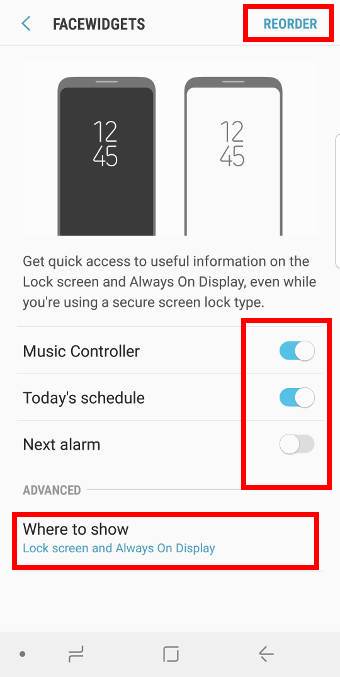This screenshot of the website features several key elements and design components. At the top, there is a faded blue arrow pointing to the left, adjacent to the word "FACEWIDGETS," which is written in black capital letters. To the right, there's a red-bordered rectangle with a white interior, containing the word "REORDER" in the same faded blue color as the arrow.

Beneath this section, a white background showcases two cell phones placed side by side, although their bottom parts are cut off. Each phone has a gray border: the left phone displays a black screen with digital numerals "1-2" and "4-5," while the right phone shows a white background with the same gray numerals. 

Below the phones, a bold caption reads: "GET QUICK ACCESS TO USEFUL INFORMATION ON THE LOCK SCREEN AND ALWAYS ON DISPLAY, EVEN WHILE YOU'RE USING A SECURE SCREEN LOCK TYPE."

Following this, the words "MUSIC CONTROLLER," "TODAY'S SCHEDULE," and a rectangular on-off toggle switch appear. Below the toggle, there's a section labeled "ADVANCED."

Towards the bottom, a long red-bordered rectangle with a white interior displays the text "WHERE TO SHOW" in black. Underneath this, in blue, it reads "LOCK SCREEN AND ALWAYS ON DISPLAY."